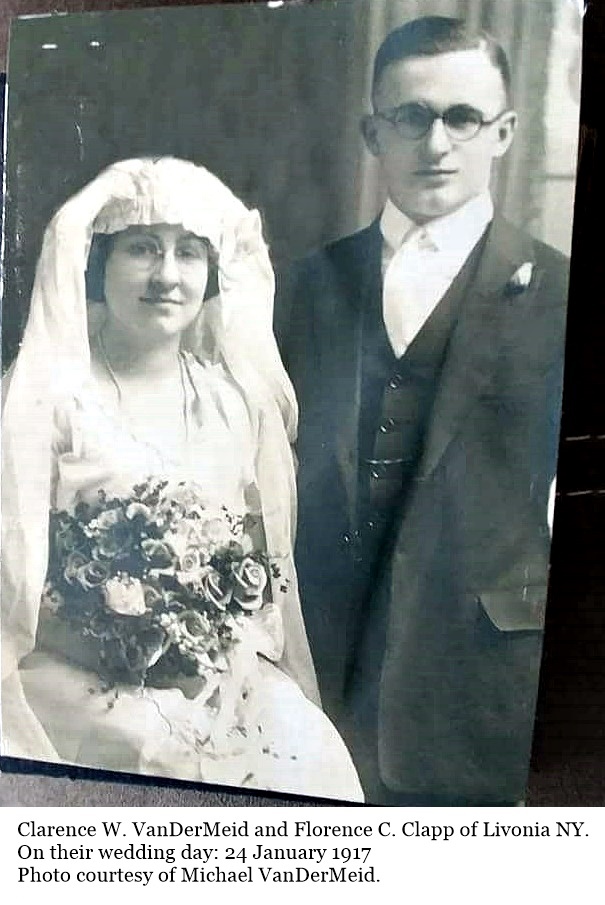This black and white photograph, dated 24 January 1917, captures the wedding day of Clarence W. Vandermyde and Florence C. Clapp of Livonia, New York. The image features the bride and groom standing indoors, with light flooding through a window behind them, suggesting a house setting. The bride, positioned on the left, is adorned in traditional wedding garb and a distinctive white headpiece resembling a kerchief with fabric draping over it. She holds a large bouquet of flowers and wears roundish glasses. Her expression is a gentle smile, reflecting the solemnity of the occasion. The groom, standing to the right, is dressed in an early 20th-century three-piece suit complete with a suit jacket, vest with four visible buttons, and a watch chain. He also sports roundish glasses and a white boutonniere, adding a dignified touch to his attire. Both bride and groom gaze calmly at the camera. Beneath the photograph, there is text stating, "Clarence W. Vandermyde and Florence C. Clapp of Livonia, New York, on their wedding day, 24 January 1917. Photo courtesy of Michael Vandermyde," all printed in black over a white background.